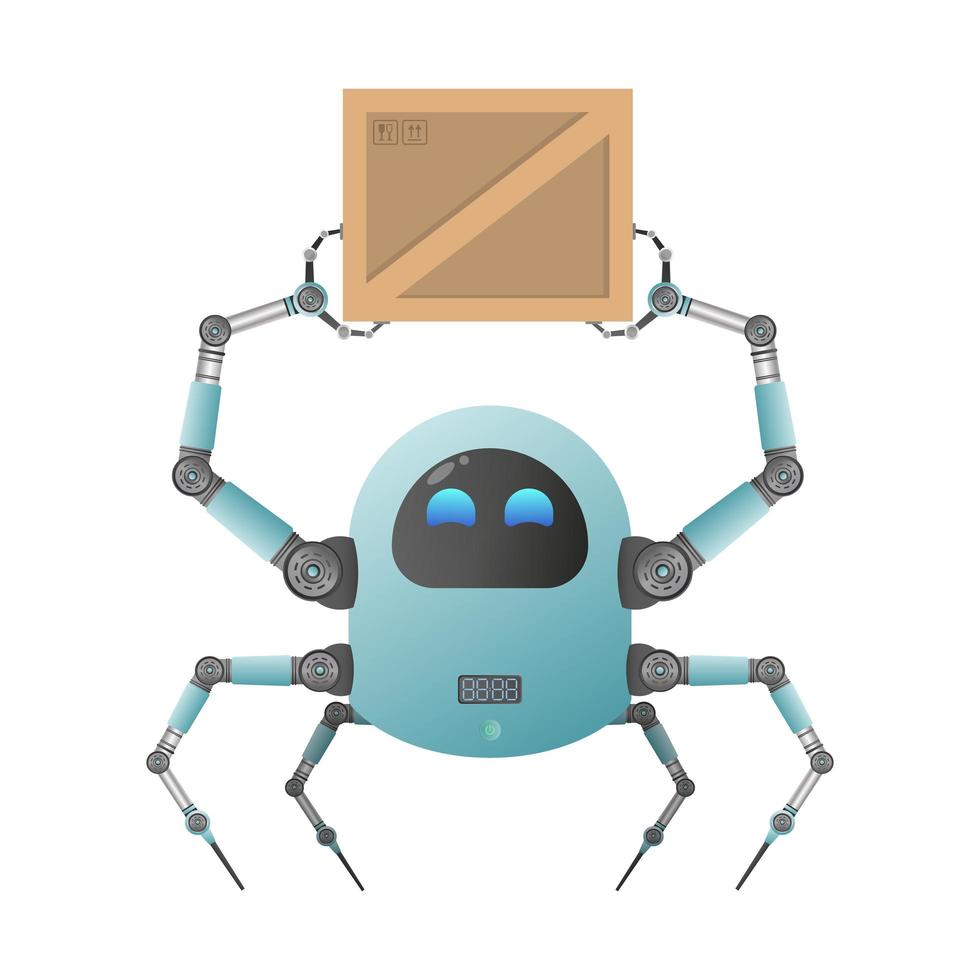This detailed image depicts a charming small robot with an egg-shaped, light blue cylindrical body. The robot has a distinct black faceplate with two blue crescent-shaped eyes, reminiscent of Eve from Wall-E, which give it a cheerful and expressive look. On its torso, it has a small black screen displaying "8888." The robot's arms stretch out to hold a large brown wooden crate above its head. This crate features packing symbols, including two wine glasses indicating fragility, and two arrows pointing upwards to signify proper orientation. 

Each of the robot's two arms, blue with black circular joints, consist of three segments: the first two segments are blue, while the final segment is silver. These segments are connected by four black circular joints per arm, providing flexibility. The robot's hands are claw-like, firmly grasping the crate. 

Its four blue legs extend from the bottom of its body, each leg segmented with three joints marked by black circular components that resemble wheels, ending in sharp, stilt-like points that stabilize the robot. The overall appearance of these legs gives an impression akin to spider legs, enhancing the robot’s quirky and industrious demeanor.